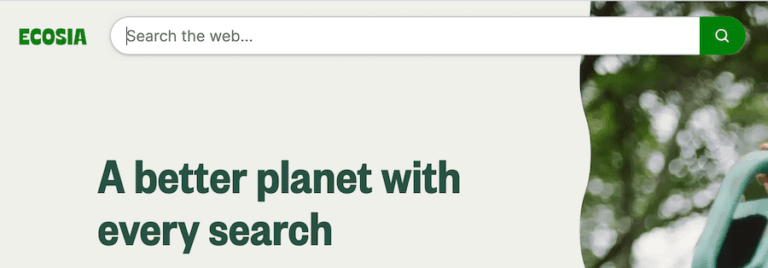This image appears to be a web advertisement or the top segment of a website for Ecosia. The background is a very light tan color, providing a soft, neutral backdrop. In the upper left corner of the image, the word "ECOSIA" is prominently displayed. Along the upper edge of the image, there is a white search bar with gray text, ending in a green section featuring a search magnifying glass icon. Adjacent to the search bar, a slogan is written in green text, reading "A better planet with every search."

On the right side of the image, there are blurry green blobs that likely represent trees, contributing a sense of environmental focus. There is an indistinct object in the right corner, and while its exact nature is unclear, it does not detract from the overall layout. The image is a horizontally oriented rectangle, suggesting it could effectively serve as a standalone advertisement, particularly appealing to environmentally conscious individuals who are interested in contributing to a greener planet through their web searches.